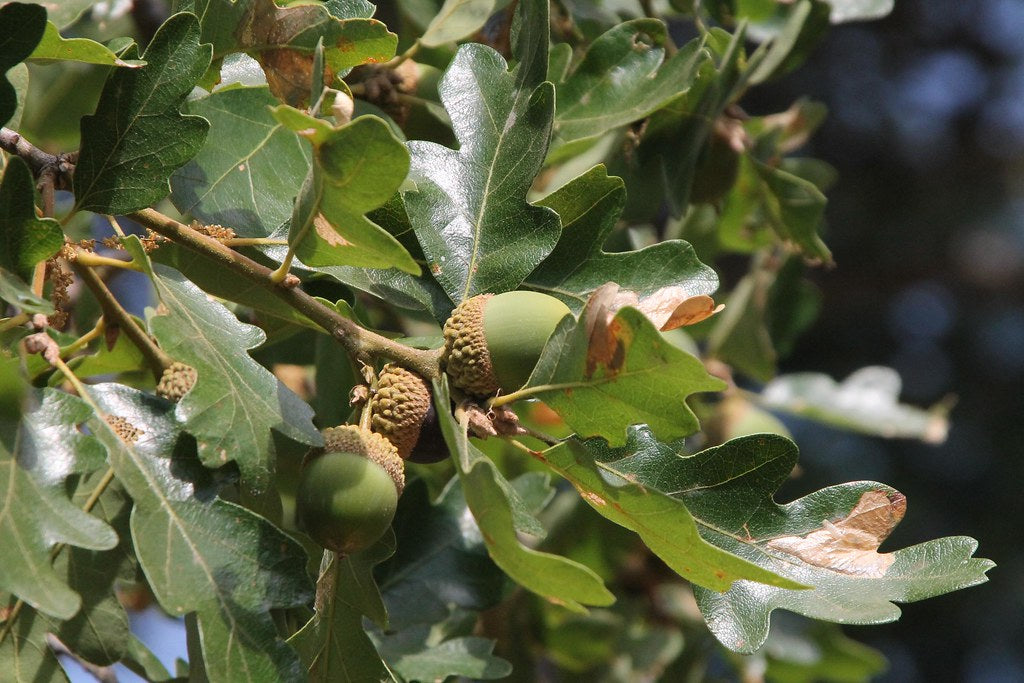This close-up photograph captures the details of an oak tree, featuring prominently green leaves with a slightly glossy, leathery texture. The leaves, in various shades of dark to light green, are arranged among brown stems. Central to the image are several large acorns, characterized by their green lower halves and distinctive brown, bumpy caps. The acorns vary in appearance, with some showing a slightly yellowish tint near the top. The composition focuses on the interplay between the acorns and the shiny green leaves, illuminated by sunlight. To the right, the image fades into a blurred, darker background, creating a contrast that highlights the vibrant foliage and acorns.